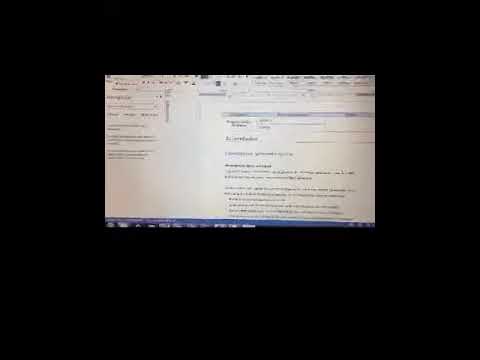The image is a very blurry, low-quality screen capture of a computer screen, possibly taken from a video camera. The primary visible elements include black text and boxes, albeit unreadable due to the poor image quality. The screen appears to display some kind of software with a toolbar, top menu, and a navigation bar at the bottom of the screen. The left side seems to contain a small paragraph of information, while the right side features a table with column headings and larger paragraphs with subheadings beneath the table. A distinct, thick, dark black border surrounds the entire screenshot, with the bottom border being particularly thicker and housing an additional blue line and symbols, which are partially cut off. This border dominates more than half of the total area of the image.